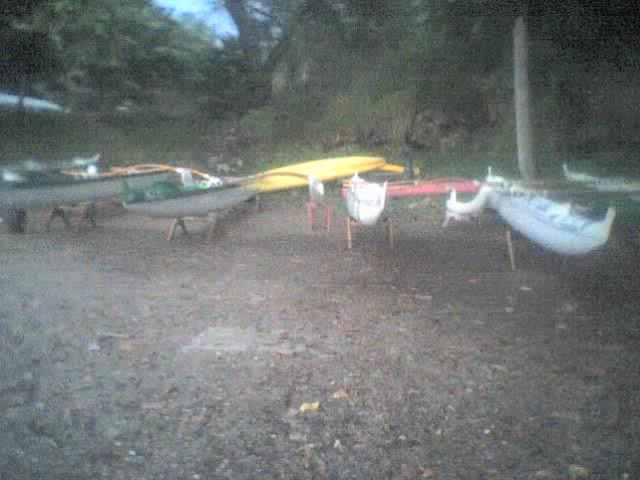In this low-resolution, grainy photo set in a campground area, several vividly colored canoes—yellow, green, white, blue, red, and multiple shades of gray—are prominently displayed on wooden pedestals, except for one yellow canoe resting on the ground. The scene has a faded appearance, with the trees and rocky, dirt-laden terrain covered by a grayish filter. The canoes are arranged centrally, creating a striking contrast against the flat, gravelly ground and the dense forest framing the backdrop. The sky peeking through the treetops hints at an afternoon setting, contributing to the overall rustic and slightly mysterious atmosphere of the image.